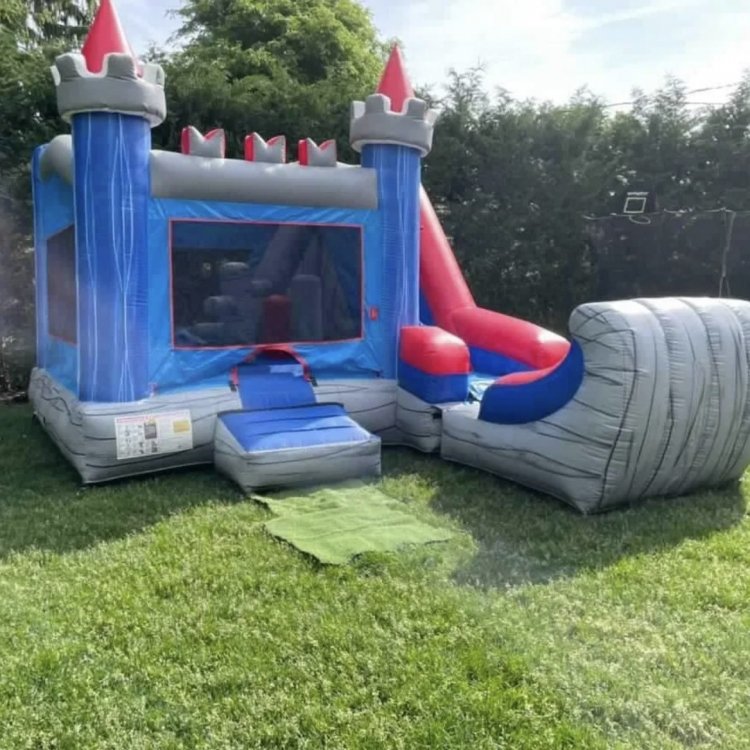The image captures a vibrant backyard scene featuring a large, inflatable bounce house designed to resemble a medieval castle. Set on lush, well-maintained green grass, the blue castle with red-tipped turrets stands prominently. The structure includes silver accenting at the top and bottom, as well as a slide extending down the right side with red railings and a silver catching area at the bottom for safety. The bounce house, surrounded by a gray-accented base, features a screened enclosure around the main play area and an inflated step for entry. In the background, a dense wall of trees frames the scene, adding a naturalistic element to the photorealistic image illuminated by natural light.